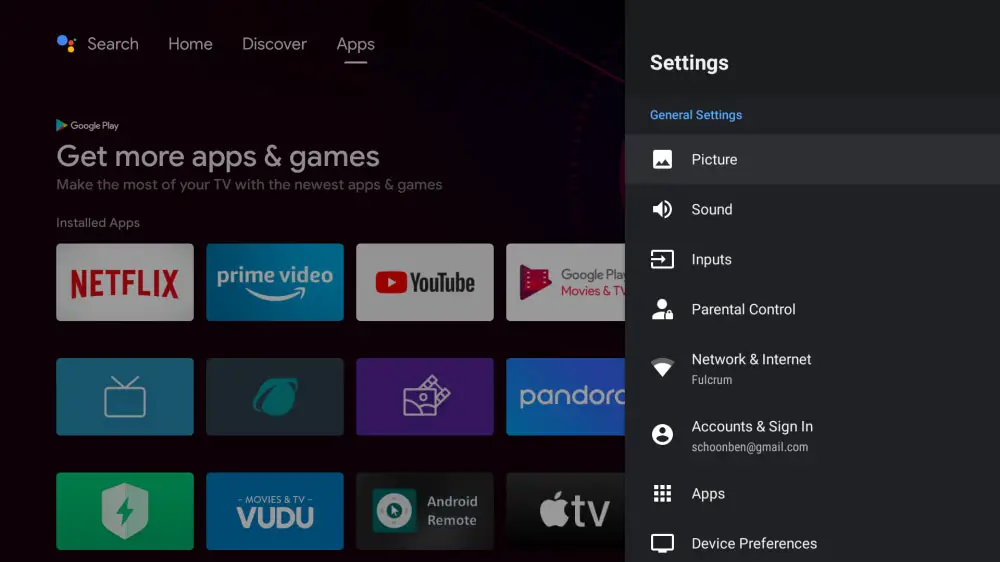The image displays a settings page of what appears to be a smart TV. At the top, it prominently features the title "Settings." Below this heading, there's a "General Settings" section that offers several options:

1. **Picture** - Represented with a picture icon.
2. **Sound** - Indicated with a sound icon.
3. **Inputs** - Shown with a screen and an arrow pointing to the right.
4. **Parental Controls** - Illustrated with the outline of a person and a lockbox.
5. **Network & Internet** - Depicted with a WiFi symbol.
6. **Accounts & Sign-In** - Lists an email address with the outline of a person.
7. **Apps** - Displayed with an icon of multiple white dots.
8. **Device Preferences** - Represented with a device screen icon.

Underneath the "Device Preferences" section, additional sections are visible:

- **Search**
- **Home**
- **Discover**
- **Apps**

In the "Google Play" section, the text "Get more apps and games" is shown, along with the message "Make the most of your TV with the newest apps and games." Below this message, there is a list of installed apps along with their colorful icons. These include popular apps such as:

- Netflix
- Prime Video
- YouTube
- Google Play
- Android Remote
- Apple TV
- Pandora
- Movies and TV
- Vudu

The text labels are primarily in grey and white, providing a clear contrast against the colorful app icons. The overall layout and content strongly suggest that the interface belongs to a smart TV.